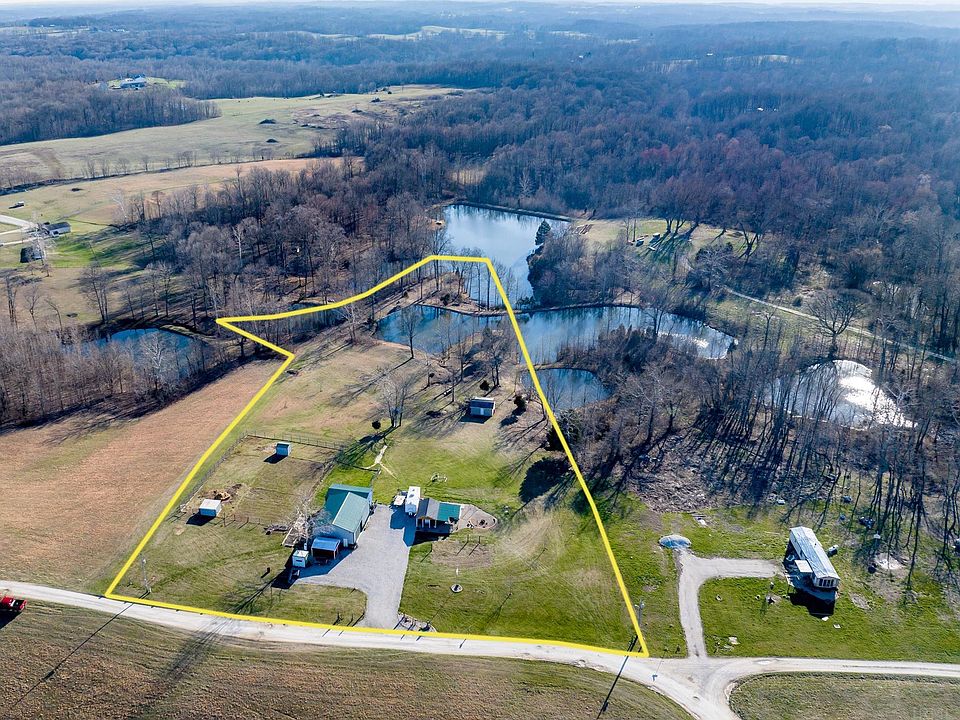This aerial view captures a diverse landscape featuring a mix of grasslands, pastures, and wooded forest areas, likely photographed in fall or early spring as most trees appear bare. Central to the image is a plot of land highlighted by a yellow boundary, which intriguingly resembles the shape of a bird's head or a duck. This delineated area encompasses a house with a tin roof, a large barn, several outbuildings, and a spacious driveway. Notably, this section contains multiple small ponds, suggesting the possibility of a fish farm. Surrounding the highlighted property are expanses of grassy areas, a network of roads, and additional bodies of water. The foreground displays mostly leafless, tall, skinny trees, while the background reveals more vibrant greenery and dense forested regions.